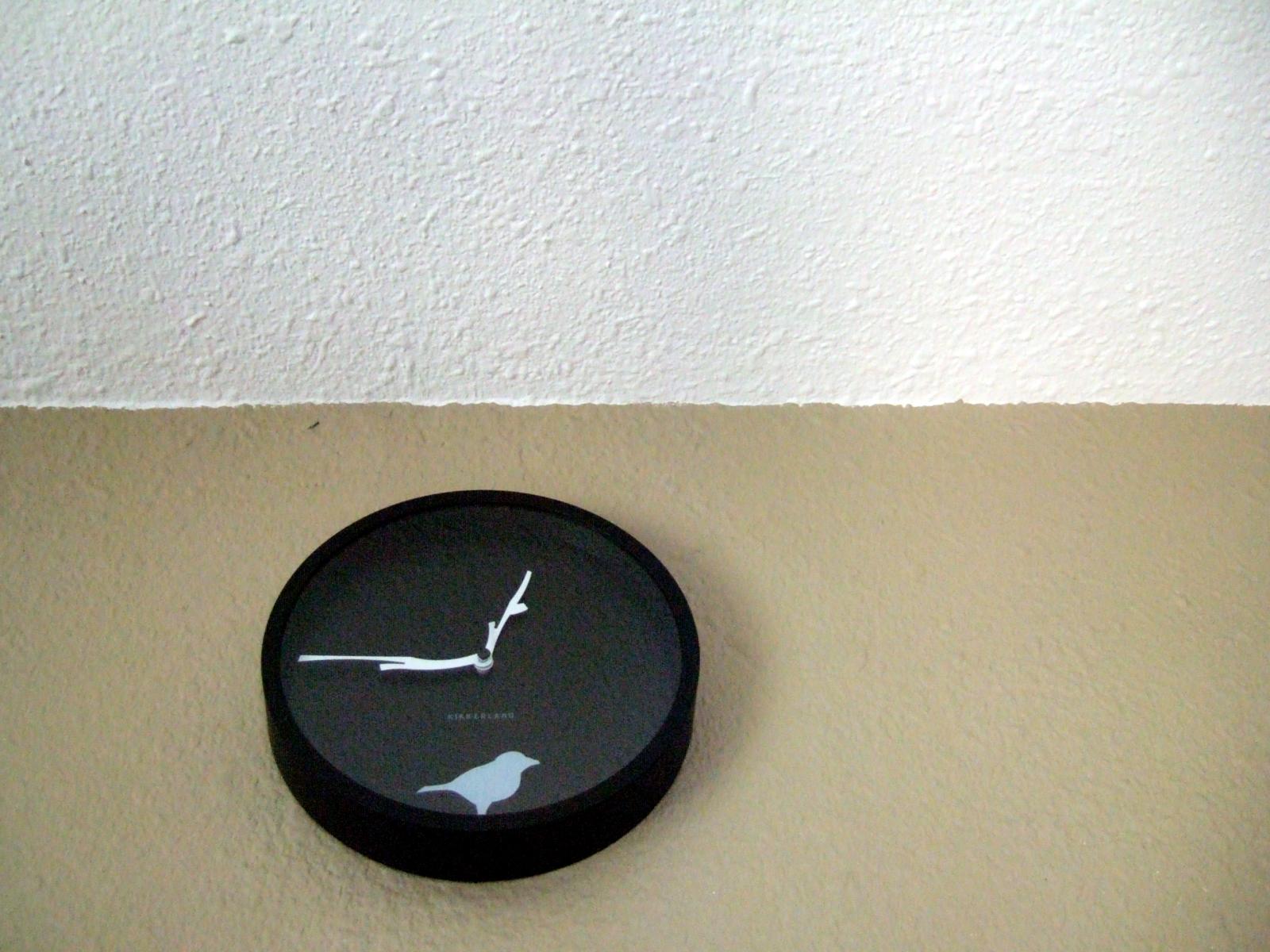This photo captures an upward view of a round, black wall clock situated near the top of a tannish, popcorn-textured wall. The ceiling, also covered in a white popcorn texture, is prominently visible, emphasizing the intersection where the ceiling paint slightly overlaps onto the wall, suggesting painter's tape wasn't used during painting. The clock, though small, has a thick black frame and lacks numerical markers. Its hour and minute hands are designed to resemble branches, adding a touch of nature-inspired detail. At the center bottom of the clock, a small bird motif is visible, enhancing its unique aesthetic. Additionally, small white writing is present below the hands, contributing to the clock's distinctive design.